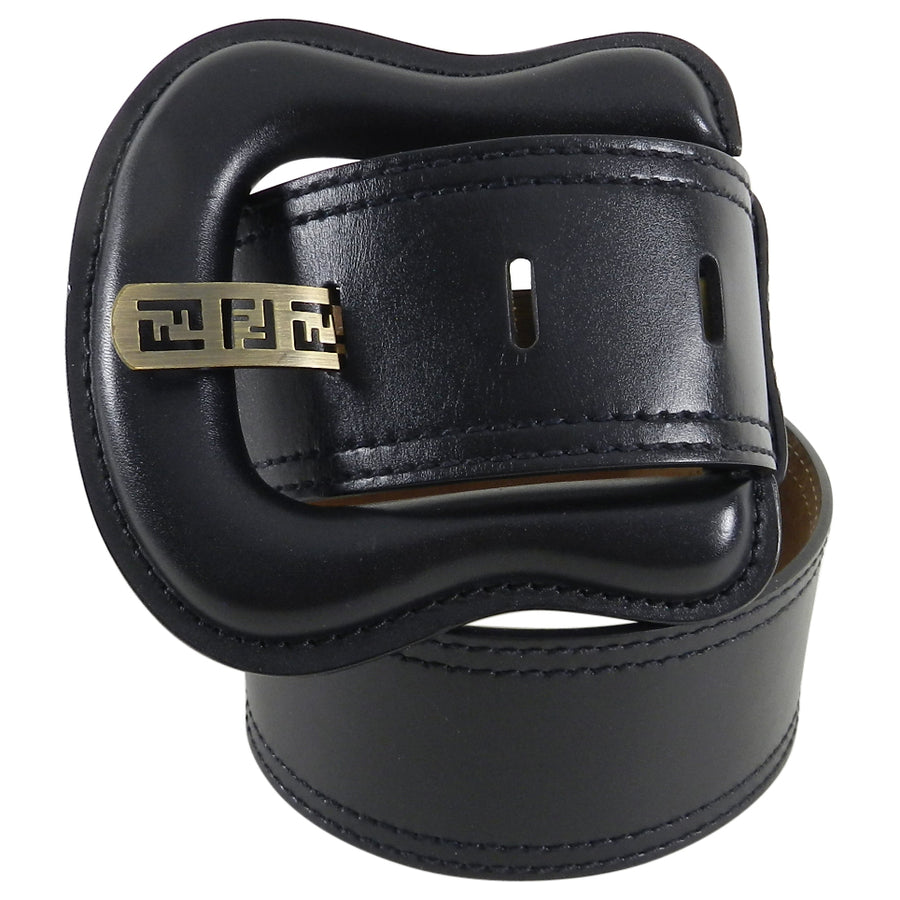This close-up photograph features a high-quality, black leather belt intricately coiled into itself, resembling a snake. Set against a pristine white background, the belt's glossy, smooth texture is highlighted. Notably, it sports double rows of seams and reveals a brown underside on its right side. The buckle, prominently displayed at the top of the coiled belt, is notable for its elongated stab and hole portions, which deviate from the traditional round shape, instead adopting an oval design. The brass-colored metal element of the buckle, richly decorated, features a unique pattern of two interlocked F's, one upright and one inverted, adding a sophisticated and distinctive touch. There are no other objects or text in the image, emphasizing the belt as the focal point, indicative of a stock photo likely intended for a clothing website.